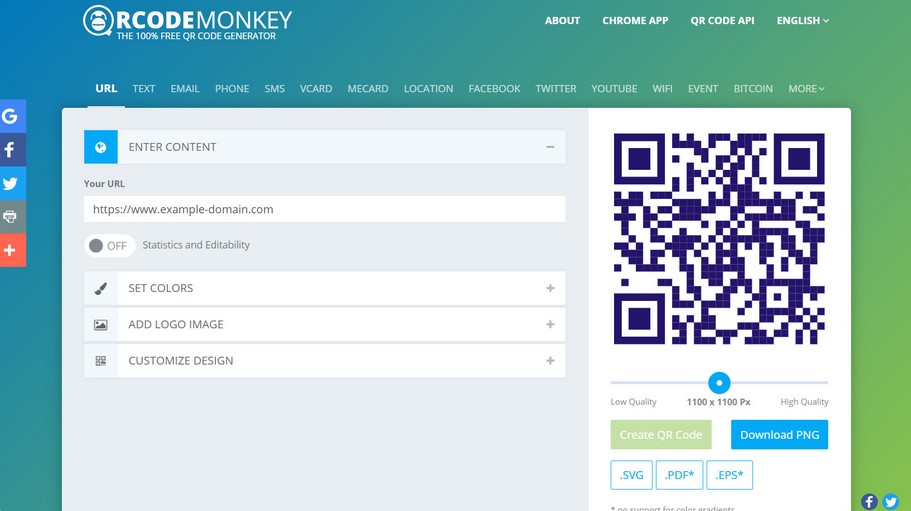The image depicts a sign-up or splash page for a service called "R-Code Monkey," a 100% free QR code generator. The brand logo and name, "R-Code Monkey," are prominently displayed on the upper left corner of the page. 

The left sidebar features icons for Google, Facebook, Twitter, printing, and a generic plus icon housed within a red square. Across the top header on the right are navigation options labeled "About," "Chrome App," "QR Code," "API," and "English," with the latter indicating a dropdown menu.

The core section of the page displays a series of selectable tabs running horizontally above the main content area. These tabs include URLs, which is currently highlighted, as well as options for text, email, phone, SMS, Vcard, MiCard, location, Facebook, Twitter, YouTube, WiFi, Event, Bitcoin, and more (with an associated dropdown).

On the left side of the main content area, there's an input box titled "Enter Content," instructing users to input a URL in the format "https://www.example-domain.com." Below this input field are a gray toggle button for "Statistics and Editability," a paintbrush icon for "Set Colors," a picture icon for "Add Logo Image," and a design icon for "Customize Design."

To the right, the main content area exhibits a live example of the QR code being generated. Users can adjust the quality of the QR code with a slider, ranging up to 1100 by 1100 pixels (PX). Below this, a "Create QR Code" button is visible but not yet selected, indicated by its light green background. Adjacent to it is a "Download PNG" button in white font against a blue background. Beneath these buttons are three further download options in white boxes labeled .svg, .pdf (marked with an asterisk), and .eps (also marked with an asterisk).

The bottom-right corner of the page contains two social media icons for Facebook and Twitter. The overall background of the page has an ombre gradient transitioning from deep sky blue to light green from left to right. No other text is present.